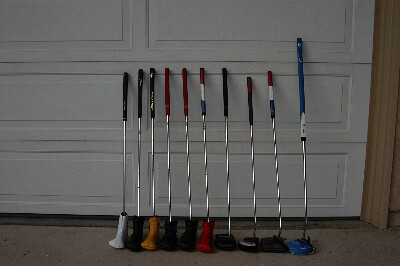This photograph depicts a collection of ten golf clubs neatly lined up on a concrete driveway, leaning against the white, multi-paneled surface of a closed, two-car garage door. Each club head is protected by a colorful sock, with hues including white, black, yellow, red, and blue. The clubs are of various types, suitable for different golfing situations, such as drivers, woods, and putters. Notable is the variety in their handles, exhibiting shades of black, red, white, and blue. The setting is dimly lit, highlighting both the clean lines of the white garage door and the detailed, vibrant socks on the club heads. To the right of the garage door, a piece of brown wood is visible, adding a subtle contrast to the scene. The clubs are arranged vertically, with their heads resting on the concrete, presenting a well-cared-for appearance of the golfing set.